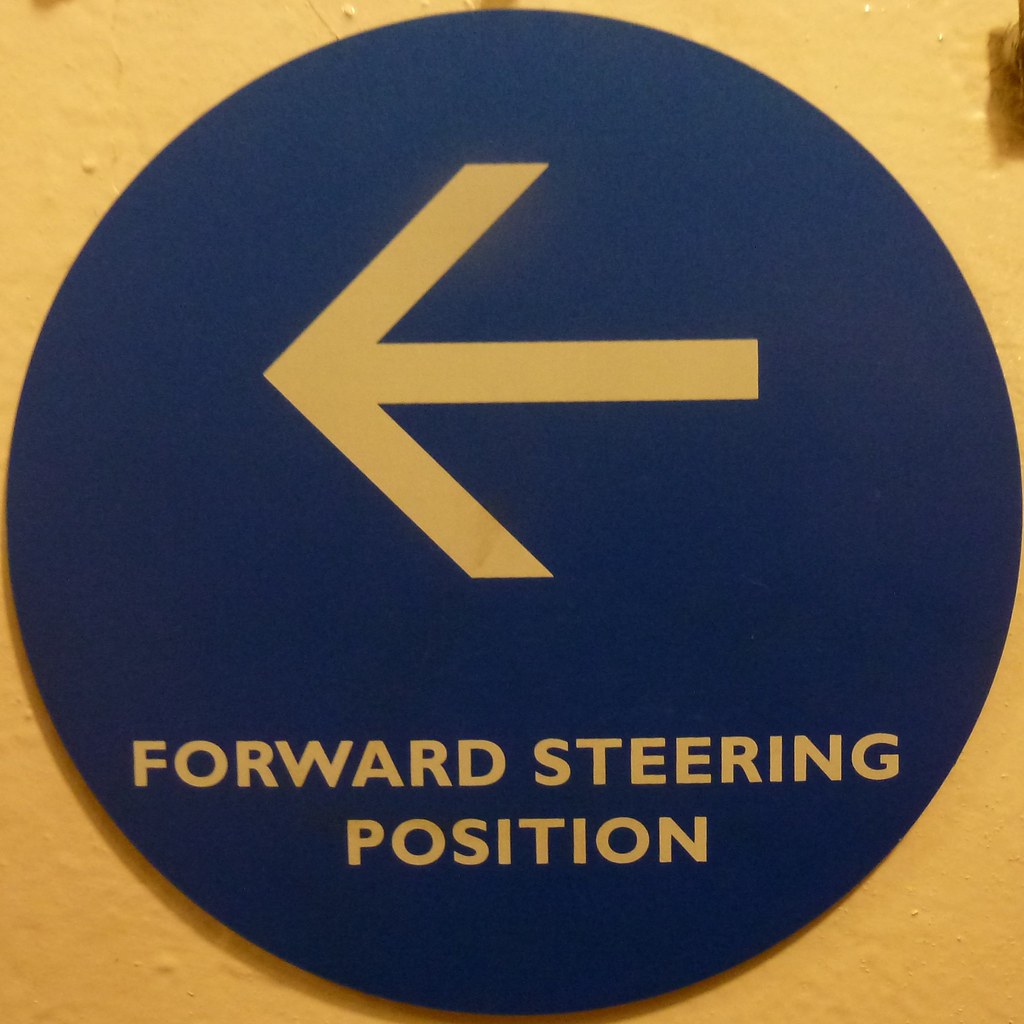The image is a close-up color photograph of a circular blue sign with a white arrow pointing to the left and white text underneath that reads "Forward Steering Position" in two lines. The sign is centered in the image and affixed to a yellow wall that appears to be made of metal, evidenced by its dimply texture. The sign's bold print and directional arrow are prominent features. In the upper right corner of the photograph, there's a small shadow cast by an indistinguishable object. The thick, institutional-style paint on the wall indicates it might be outside, although the close-up nature of the photograph makes it difficult to be certain about the exact setting.